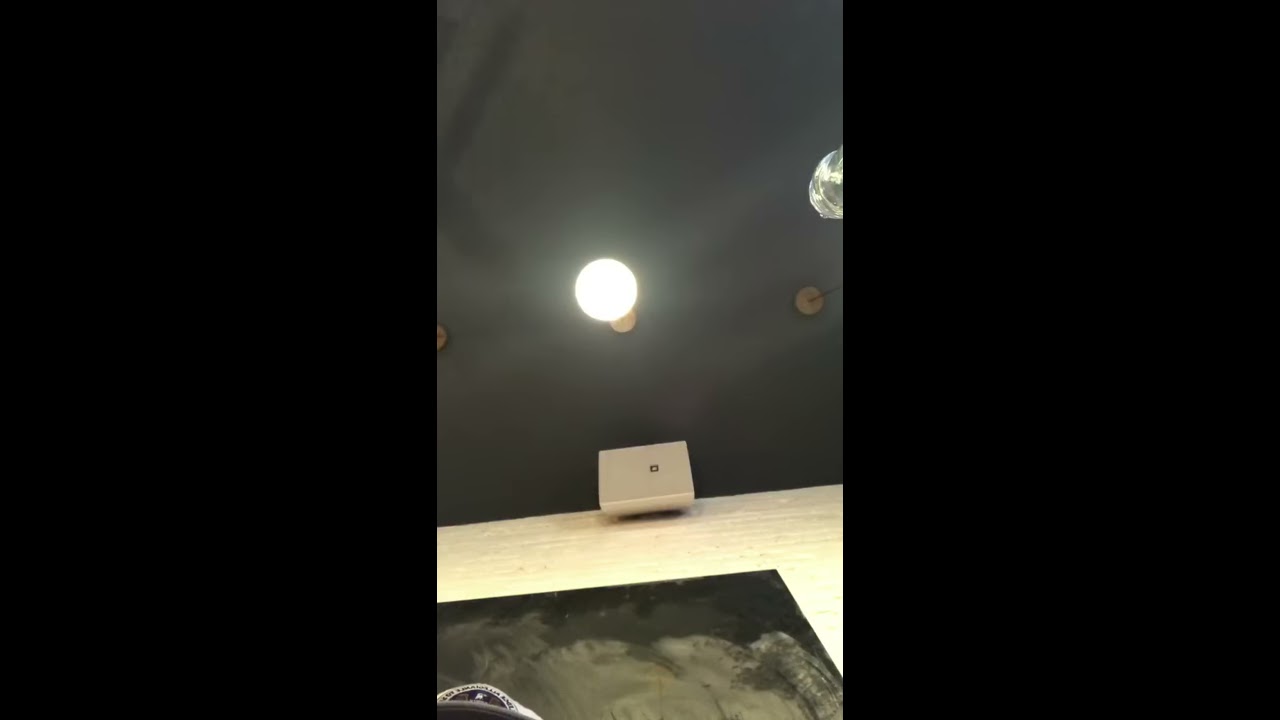The photograph, captured in portrait orientation, shows an intricately designed scene from floor level looking up towards the ceiling. The central feature is a glowing light bulb hanging from an artsy light fixture against a dark or black ceiling. The image has significant black borders on the left and right sides, making the actual viewable area smaller in comparison. Adjacent to the ceiling is a wall, which appears to be tan or painted in a light beige tone.

Where the ceiling meets the wall, a gray speaker is positioned. Moving down the photo, the wall continues to the bottom edge where it meets a piece of wall art. This art appears to have a dark canvas with gray or brown smudges, though the specific details are indistinct. Additionally, near the speaker, there is mention of a round, silvery object on the top right side, suggesting a modern aesthetic. At the lower portion of the wall, there appears to be a wood area containing various items, complemented by another silvery object and a beige device resembling an old alarm clock with a black dot centrally placed within it.